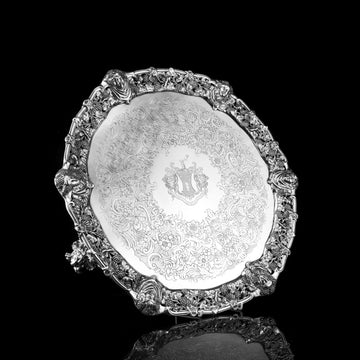The black and white photograph captures an intricately designed, oval-shaped metallic plate or serving tray set diagonally against a black background. Central to this ornate piece is a faded coat of arms or emblem, possibly etched or engraved, that hints at its age and historic significance. Surrounding this central emblem is a lighter gray, possibly ceramic or stone, area that appears worn, with faint remains of what might have been painted decorations, now faded with time. Encircling this central section is an elaborately textured and patterned metallic border that reflects light, suggesting the presence of raised engravings or possibly even jewels, giving the rim a heavy and sparkly appearance in the monochromatic photo. The plate's exquisite detailing and partial reflection at the bottom of the image highlight its craftsmanship and display setting.